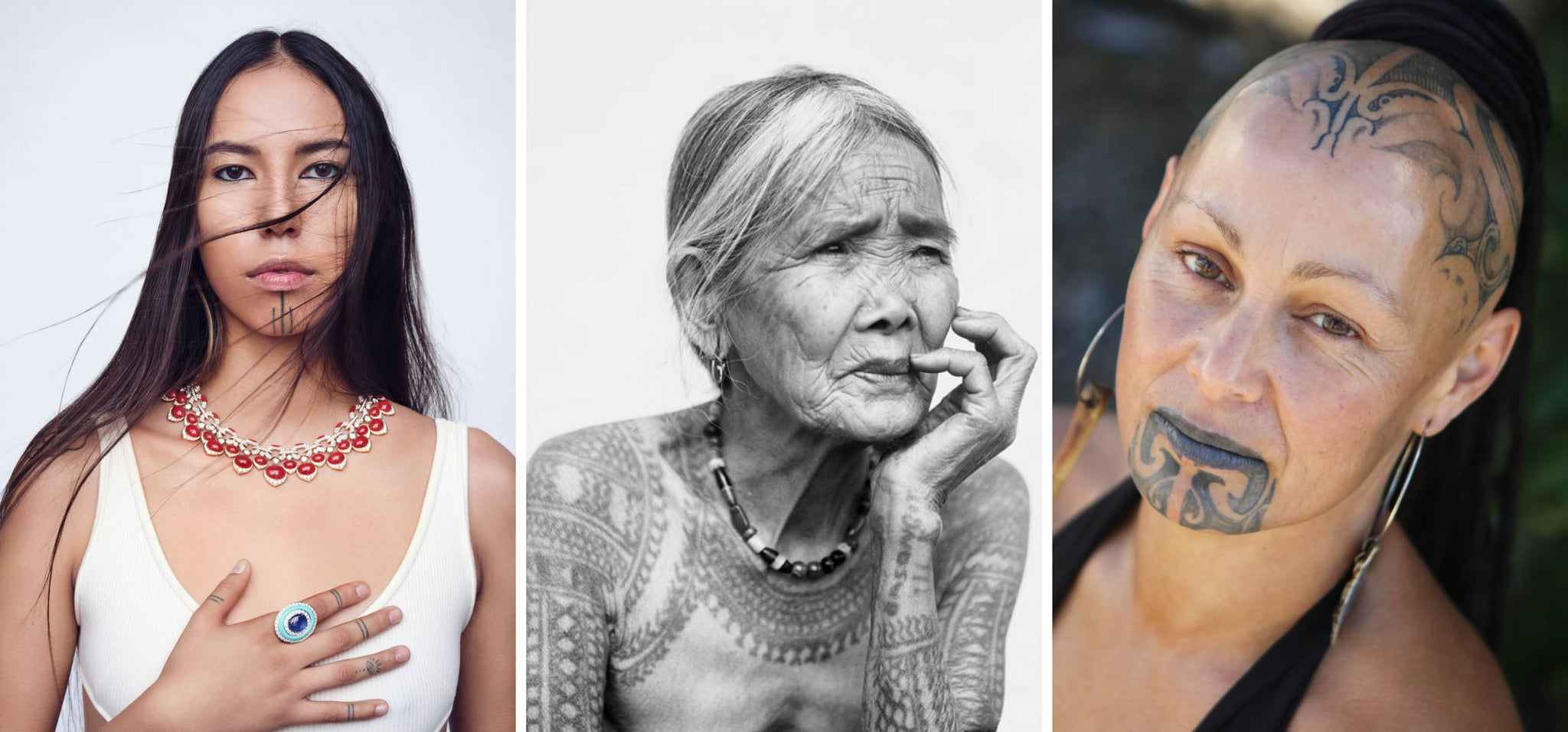The image presents three separate photographs of distinctively tattooed women arranged in a row. On the left, a young woman with long, straight, dark hair and dark eyes stands with her hand held against her chest, adorned with a large blue ring. She wears a white tank top and a striking red and gold necklace. Intricate tattoos featuring horizontal black lines mark each of her fingers, accompanied by three vertical tattoos under her mouth reaching toward her chin, which lend an appearance of Native American heritage. In the center, an elderly woman gazes into the distance in a black and white photograph. Her deeply wrinkled face and long, pulled-back gray hair suggest a life rich in stories. She sports a beaded necklace and extensive body art, with tribal tattoos covering her shoulders and arms. One hand is thoughtfully placed near her face, displaying her cultural ornaments and body art. On the right, a bald woman looks directly into the camera, her head adorned with symmetrical tribal designs in dark blue and black that flow from her scalp down to her lips and chin. She wears metallic silver hoop earrings and what appears to be a black top. The tattoos and her direct gaze convey a bold, confident presence. The background of all photos is uniformly blurred in shades of gray, ensuring that the focus remains on the women's unique appearances and expressions.